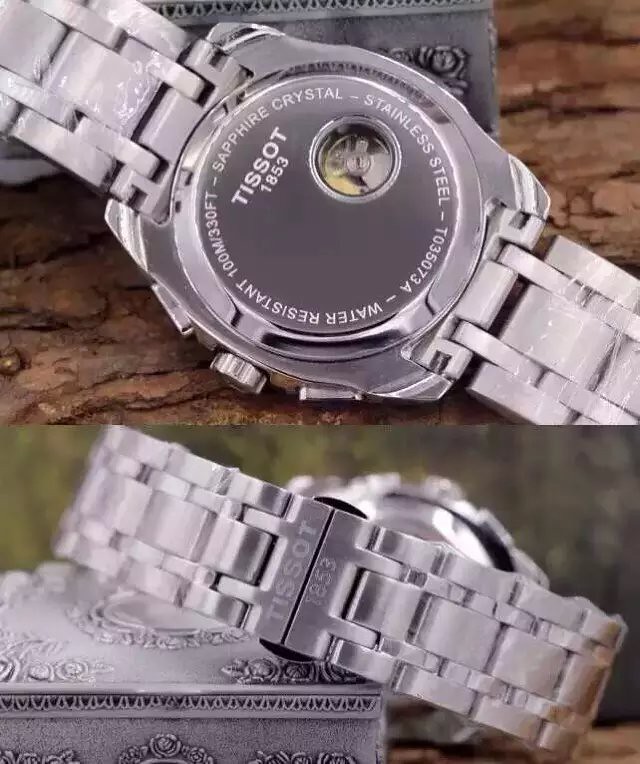This color photograph, likely intended for an advertisement, captures a sophisticated men's wristwatch in an indoor setting. The primary focus is a sleek silver watch with a metallic band that wraps around the top section of the image. The watch is flipped to display its backside, revealing detailed inscriptions that include "Tissot 1853," "Sapphire Crystal," "Stainless Steel," and "Water Resistant." The numerical codes "T035.407A" and "100M/330FT" are also visible. In the lower section of the photo, there's a close-up of the bottom part of the band, which also bears the "Tissot 1853" engraving. The band rests gracefully on a small, elegant silver jewel box, highlighting the luxury and meticulous craftsmanship of the timepiece.